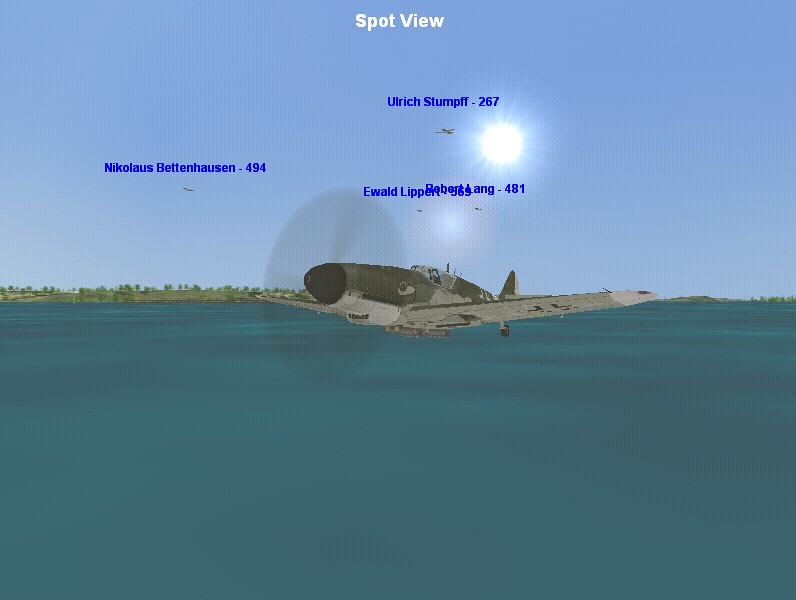This computer-generated image depicts a detailed scene featuring an airplane in flight. The sky is a soft, light blue, dominated by a glowing white sun positioned centrally. At the top of the image, the title "Spot View" is prominently displayed. Names written in blue intermingle subtly with the sky's hue.

Below the sky, dark teal green waters stretch out towards the horizon. In the distance, patches of green land emerge, adding depth to the setting. The airplane, composed of various shades of gray, has a sleek, elongated body with a pronounced dark gray nose. Its two wings are extended, and its landing wheels are visible. The cockpit appears clear, providing a transparent view inside. Interestingly, the airplane's nose is artistically adorned with an eye, and beneath it, a mouth-like feature, giving it a whimsical, anthropomorphic appearance.